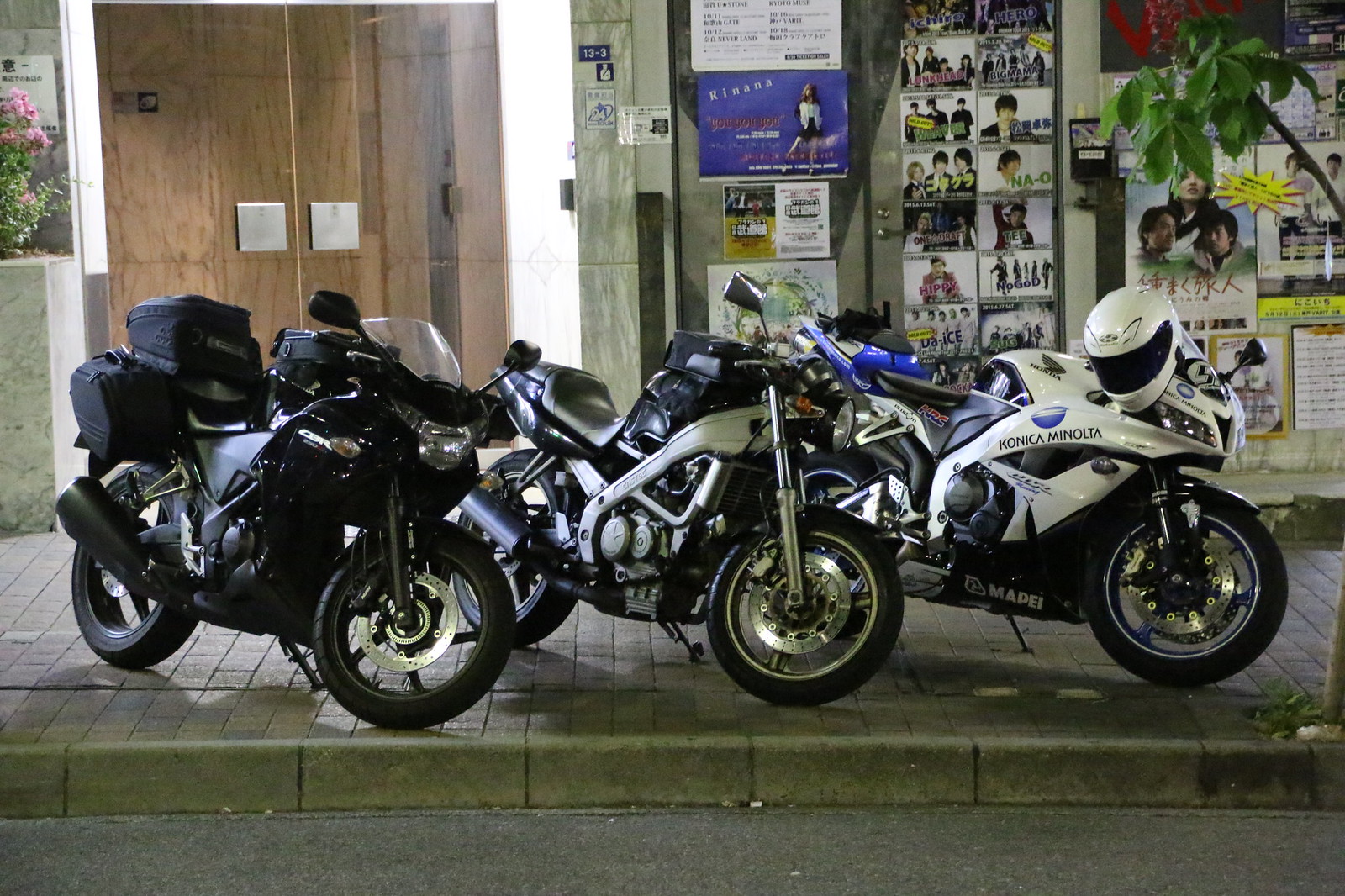This color photograph, taken at nighttime, features three sporty motorcycles parked side by side on a brick sidewalk beside a road. The motorcycles, all newer models, are positioned with their front wheels facing the street and diagonally angled to minimize obstruction. From left to right, the first motorcycle is an all-black model, the second is black with silver trimmings and a tan or gray seat, and the third is a white and blue sports motorcycle with "Konica Minolta" and "MAPEI" branding, accompanied by a white helmet on its right handlebar. 

At the edge of the sidewalk on the right is a small tree with a visible trunk at the bottom and large green leaves at the top. In the background stands a storefront with a sleek, modern appearance, featuring wooden double doors with square metal handles and large glass panels. The right side of the storefront is adorned with numerous posters and flyers depicting young Asian individuals, likely indicating an Asian location, possibly Japanese or Korean.